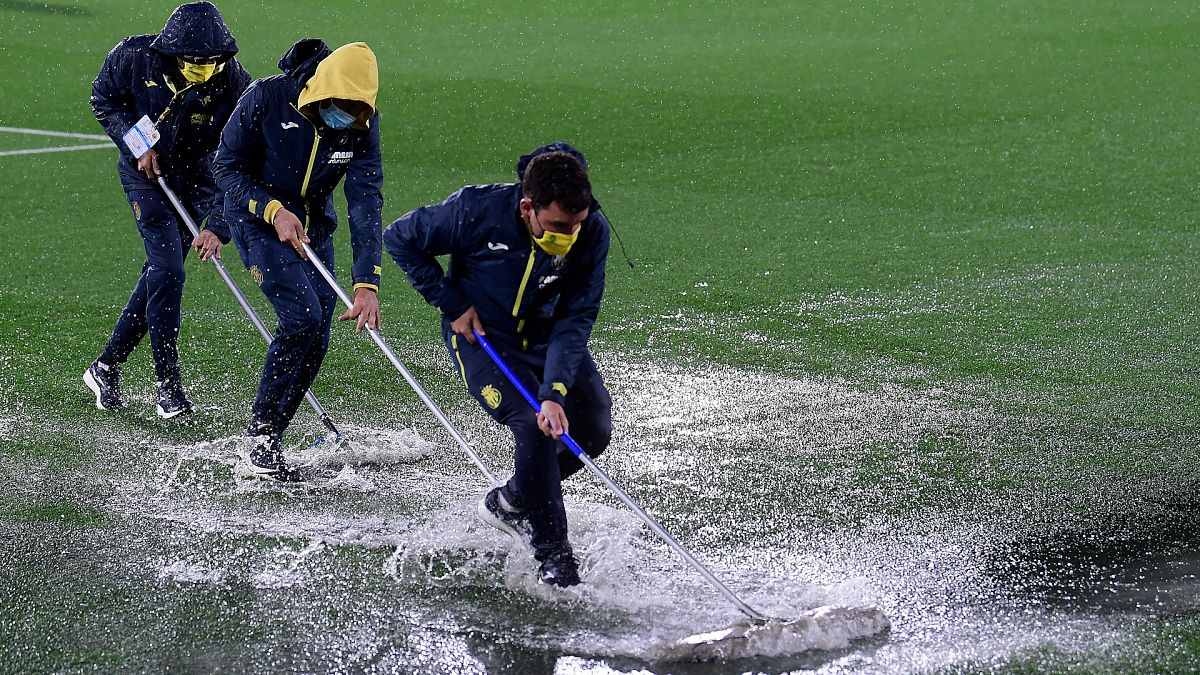The image captures an outdoor scene at a sporting event during the COVID-19 pandemic, showcasing three workers diligently clearing water from a large, grassy soccer field with squeegees. All three are dressed in dark blue tracksuits and tennis shoes, with face masks on for safety. Two of them have their yellow hoods up, while the third has his hood fallen off. They stand in a line, methodically pushing water to the side, causing splashes as they work. The workers' squeegees have differently colored handles; two are silver, and one is royal blue. The extensive green turf indicates that the field is likely well-maintained. These workers appear to be part of the assistance team responsible for maintaining the field in playable condition.